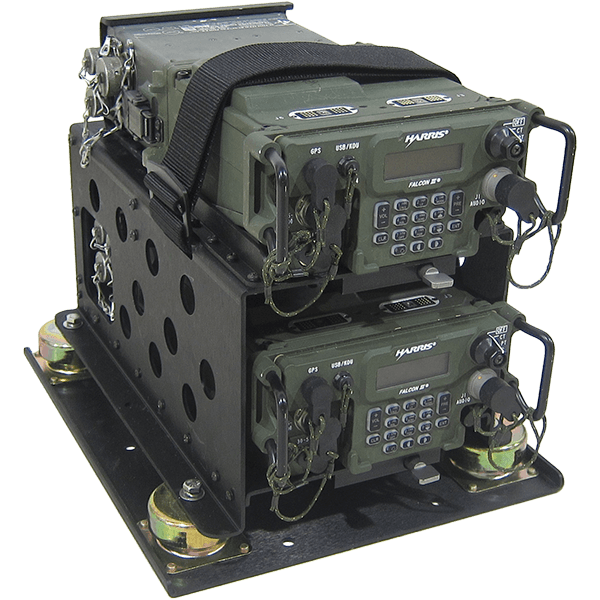The photograph shows two identical pieces of olive green military equipment housed together within a sturdy black metal case. Both machines are mounted on metal feet and are secured with a black cloth strap over the top. Each machine features a small electronic display on the front, with the brand name "Harris" prominently displayed above it. Below the display, there is a keypad resembling telephone buttons. The machinery has multiple connectors on the right-hand side, including cords and plugs, and on the left-hand side, there are rubber stoppers with attached silver chains that can be inserted into the machine. The background of the image is completely white, highlighting the robust and utilitarian design of the equipment. The entire setup hints at a possible military application, further indicated by mentions of "Harris Falcon" and "GPS," suggesting a communication or navigation-related function. The viewpoint of the photograph shows the machine from a three-quarter angle, tilted towards the bottom right-hand corner, emphasizing the layered and complex structure of the equipment.